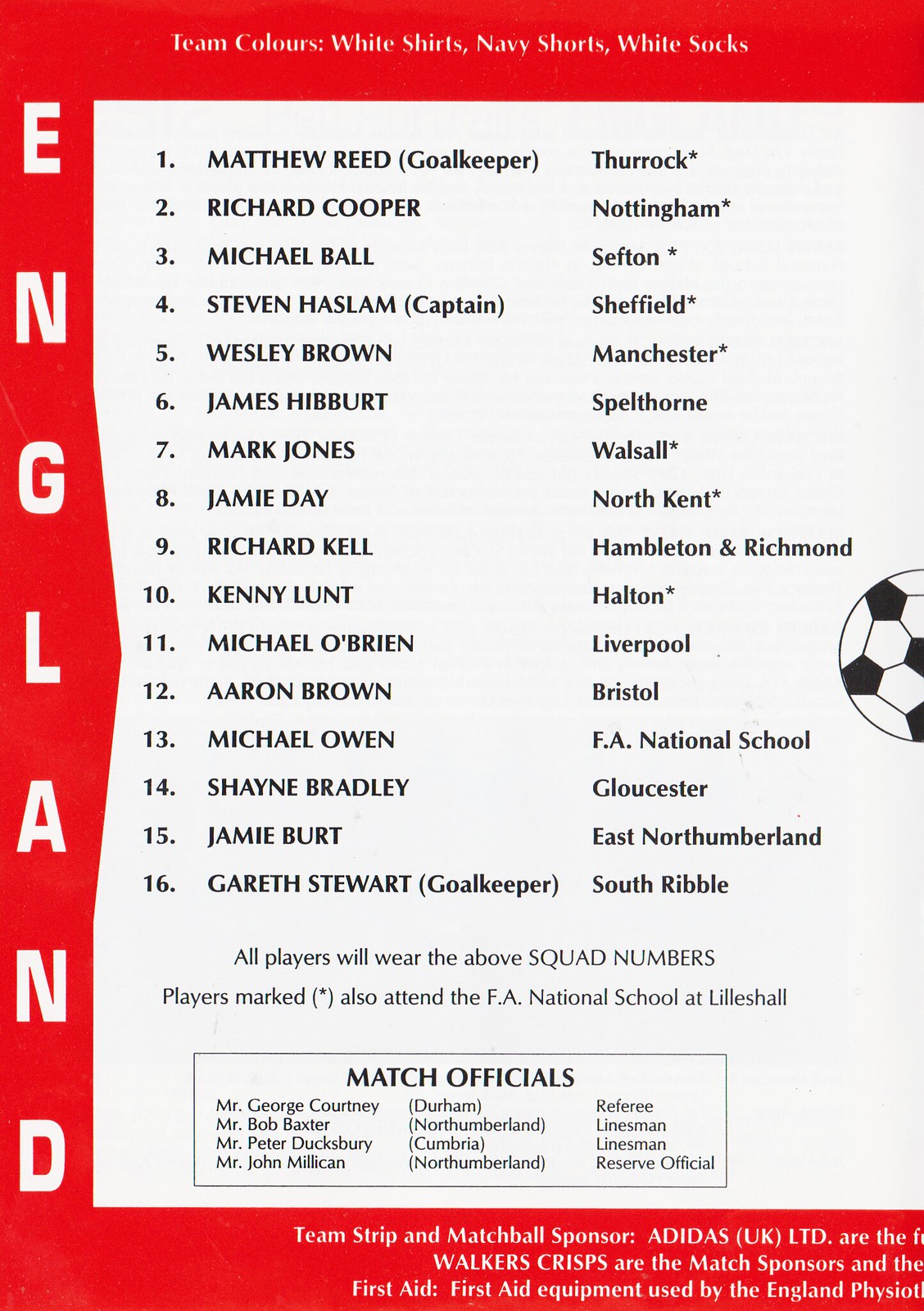This is an image of a page taken from a British football program, featuring a white background with a red border along the top, bottom, and left side. The word "England" is written vertically in red along the left margin. At the top, the text details the team colors: white shirts, navy shorts, and white socks. Following this, there is a list of 16 players, detailed from 1 to 16, along with their origins and soccer positions. The description also specifies that all players will wear their designated squad numbers, and those marked with an asterisk attend the F.A. National School at Lilleshall. Further down, a small box outlines the match officials and their origins. At the bottom of the page, sponsorship details are provided, listing Adidas and Walker's Crisps as sponsors, along with first aid information for the match.